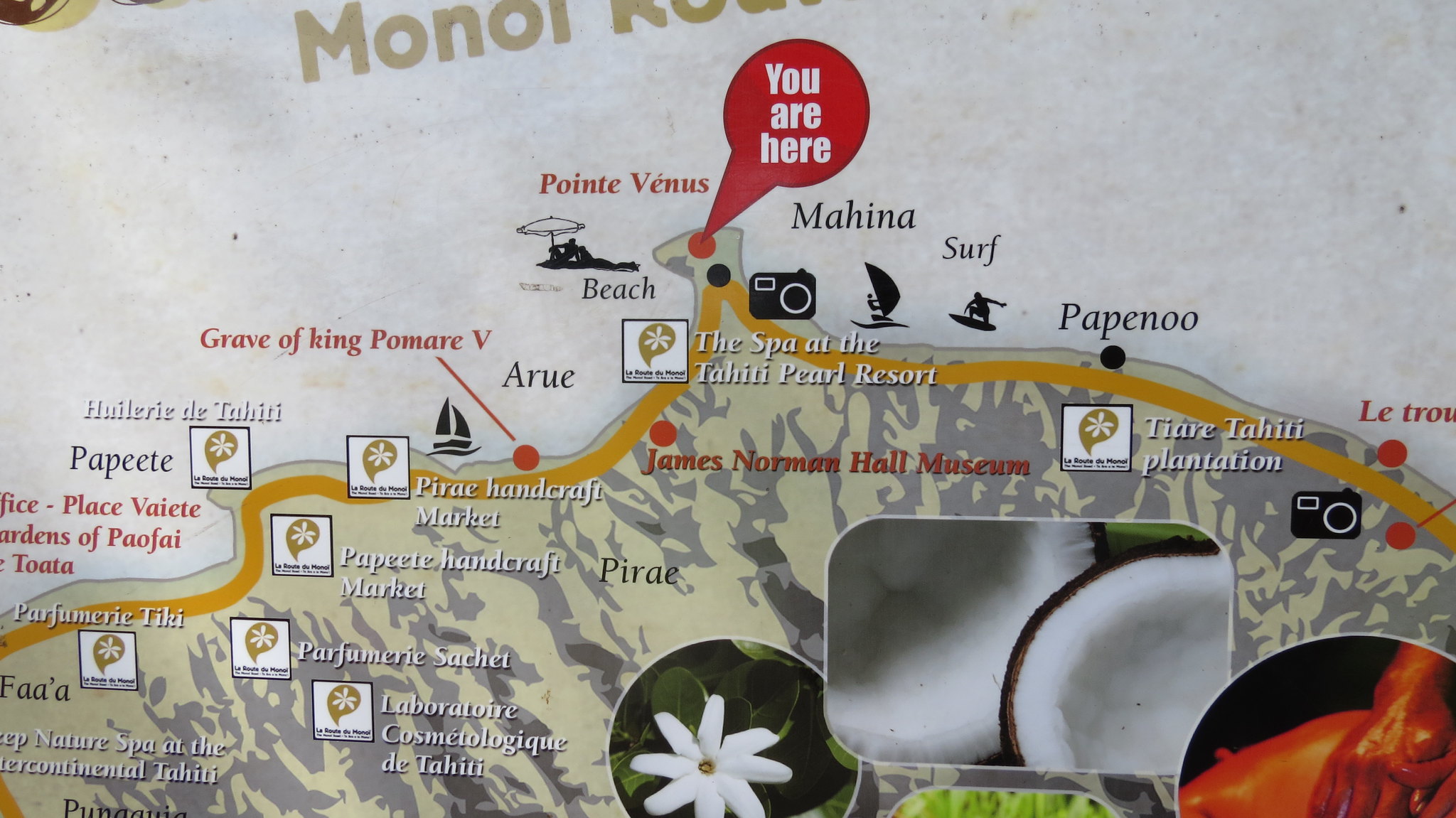The image is a detailed, color-illustrated map in landscape orientation, depicting a tropical coastline road with various points of interest. At the center of the map, in a bright red conversation bubble, the text "You are here" points to Pointe Venus beach on a small protruding island. The map is adorned with numerous icons, including a camera, a sailboat, and windsurfers, as well as symbols representing beaches, spas, and other areas to surf. A gold squiggly line meanders across the map, indicating a route with stops marked by emojis, such as a sailship and specific landmarks like the "Grave of King Pomer V." The upper half of the map features a white background with gray spots and a rippling effect on the left side, while the text "M-O-N-O-I" appears partially off-screen at the top center.

In the lower-right corner, three photographs add visual interest: a rectangular black-and-white image of a pastry and a coconut, a circular photo of a white flower with green foliage, and another circular photo, partially cropped, showing a red crustacean. The overall style combines illustration, photography, and graphic design, creating an engaging and informative guide to the coastal area's attractions.